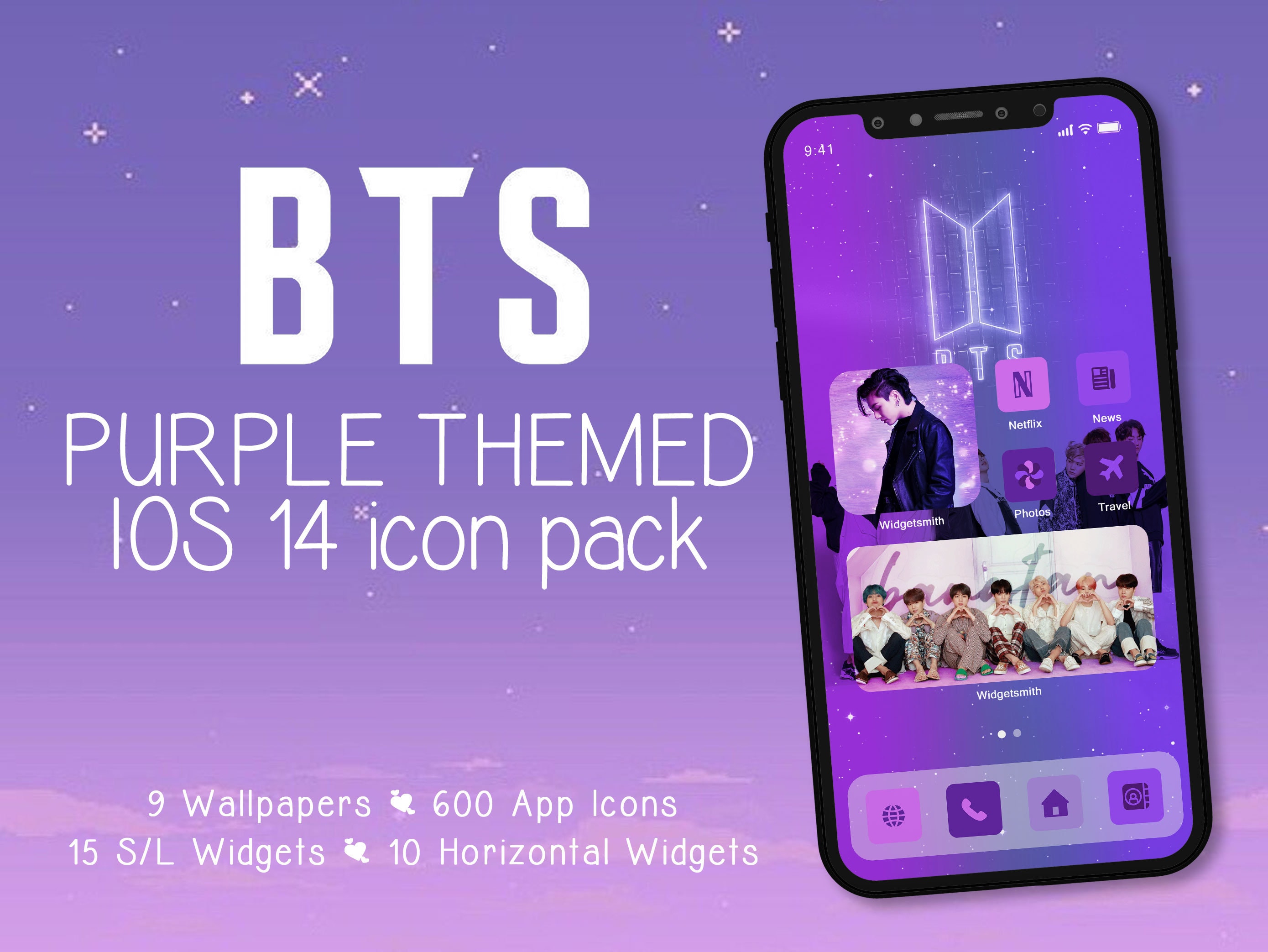The image, likely intended for a wallpaper pack advertisement, features a richly detailed, computer-generated design with a predominantly purple theme. The background transitions from a dark purple at the top to a lighter lavender hue toward the bottom, depicting a night sky with stars and clouds. On the left side, large white text reads "BTS Purple-Themed iOS 14 Icon Pack." Below this, additional information in white letters includes details such as "9 Wallpapers," "600 App Icons," "15 S-L Widgets," and "10 Horizontal Widgets," each accompanied by a small heart logo.

To the right is an iPhone showcasing the icon pack. The phone’s screen continues the purple theme with app icons visible, including Netflix and News, among others. One of the app icons features an image of a BTS member looking to his right at the ground. At the bottom of the image, there's a group of BTS members seated together. The phone's background also maintains the cohesive purplish color theme, tying the entire advertisement together seamlessly.